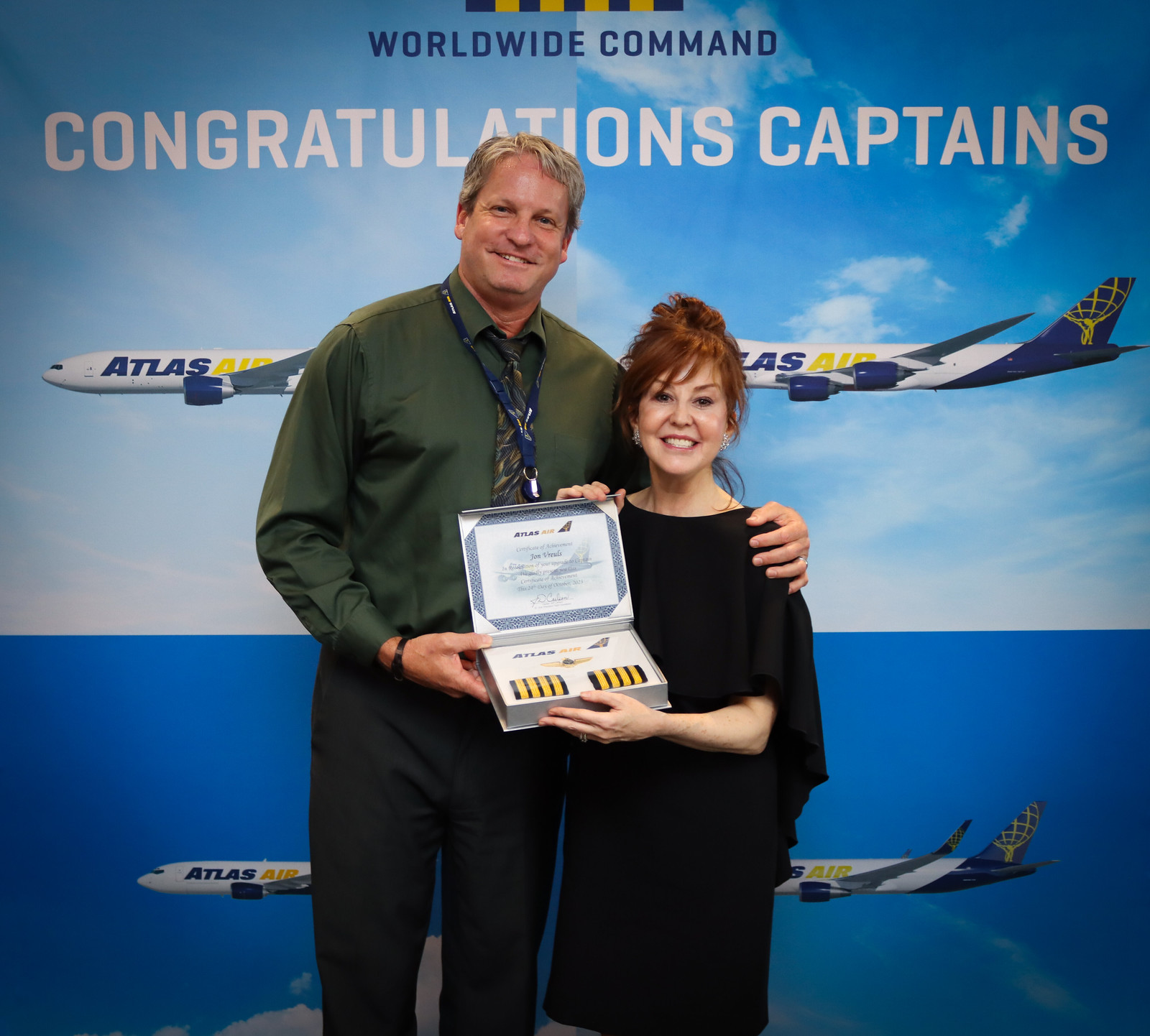In this indoor color photograph, a man and a woman are the central figures, standing side by side and posing with an award. Behind them is a banner with four images of Atlas Air airplanes flying against various colored skies. The banner reads "Worldwide Command, Congratulations Captains" in bold white type. The man, who is tall and clean-shaven, has blonde hair and wears a dark green patterned shirt with black pants. He has an ID badge around his neck, partially obscured by the award. His left arm is around the woman beside him, and both are smiling at the camera. The woman has her brown hair pinned up and wears a long black gown. They are jointly holding an open award box. The top of the box displays a certificate of appreciation from Atlas Air for "John Rolls," featuring the company’s logo and an image of an Atlas Air airplane. The bottom part of the box contains blue and yellow stripes, likely for a pilot's uniform. The scene is one of celebration and recognition, captured in a moment of shared accomplishment and joy.